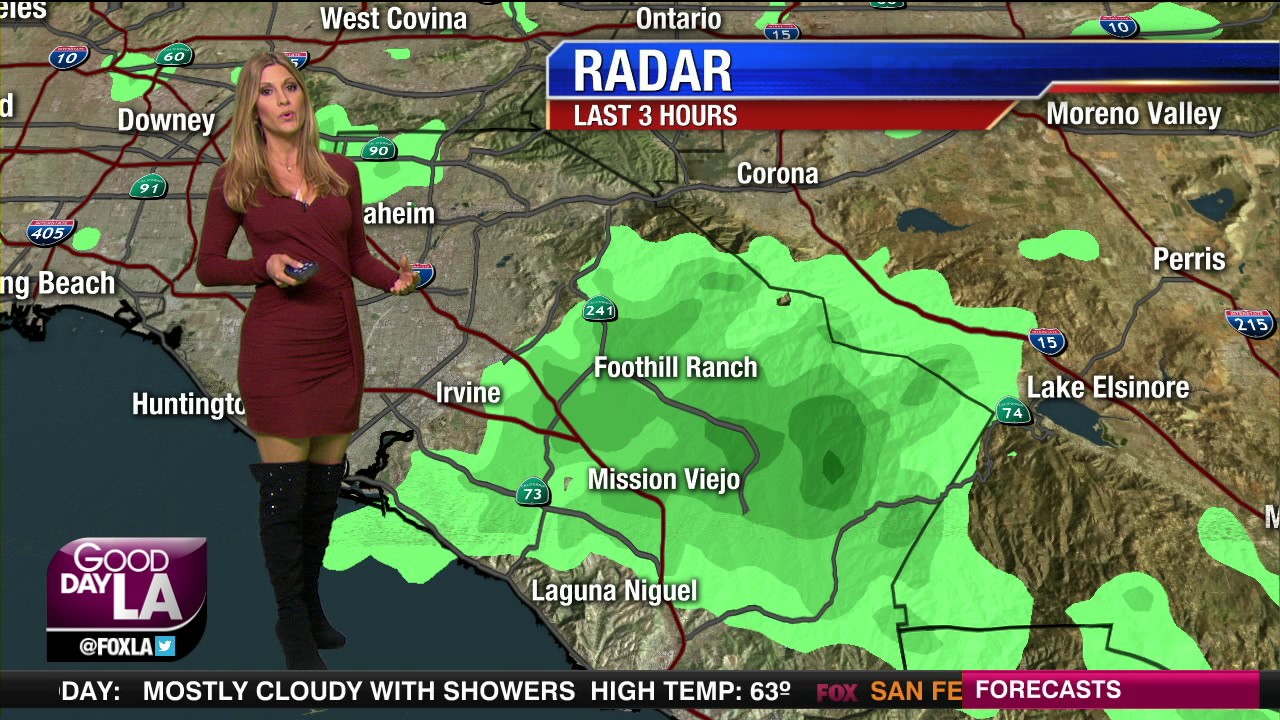In this image, a weatherwoman stands to the left of a superimposed weather map displaying radar data. She has long blonde hair and is dressed in a form-fitting dark red dress paired with black over-the-knee boots. Holding clickers in both hands, she appears to be in her 30s or 40s and points towards the left side of the screen. At the top, white letters on a blue background indicate "Radar," and below it in red, it says, "Last Three Hours."

In the lower-left corner, a purple background features the text "Good Day LA" in white, next to the Fox LA symbol. The map showcases regions likely in California, specifically Corona, Irvine, Mission Viejo, Laguna Niguel, Huntington, and Moreno Valley. A green blotch, indicating rain, is centered over Foothill Ranch, Irvine, Mission Viejo, and west of Lake Elsinore. The bottom of the screen reads, "Mostly cloudy with showers, High temperature 63," and in the right corner, in pink, it says "Forecast."